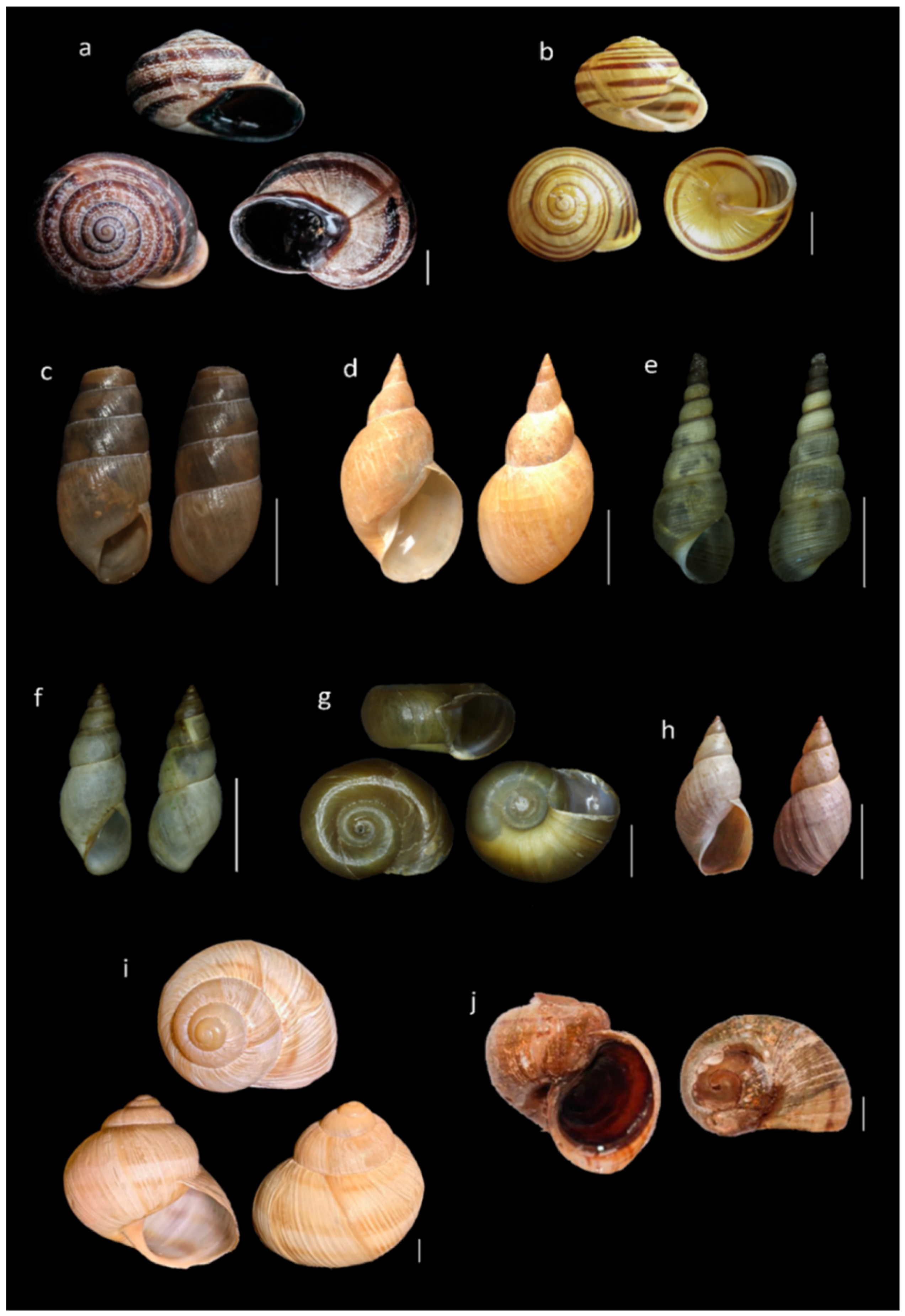This image displays a variety of seashells and snail shells arranged against a black background, each meticulously labeled from A to J. The shells vary in size, most being no larger than an inch, some as small as half an inch. In groups of three, shells A and B both feature spiral-shaped, brown, snail-like designs, suggesting they are from the same species. Shell C is a pointy, brown conch shell, while D is a similarly shaped shell but in pink. E and F mirror each other with their blue-gray conch forms. The collection grows more diverse with G, a greenish-gray snail shell, and H and I, both pink but with H being more rounded. J stands out as a thinner, more elongated, orange-brown snail shell. The shells span a spectrum of colors, primarily darker hues with some lighter variants. This vibrant assortment evokes the diverse shell fragments found along ocean shores.